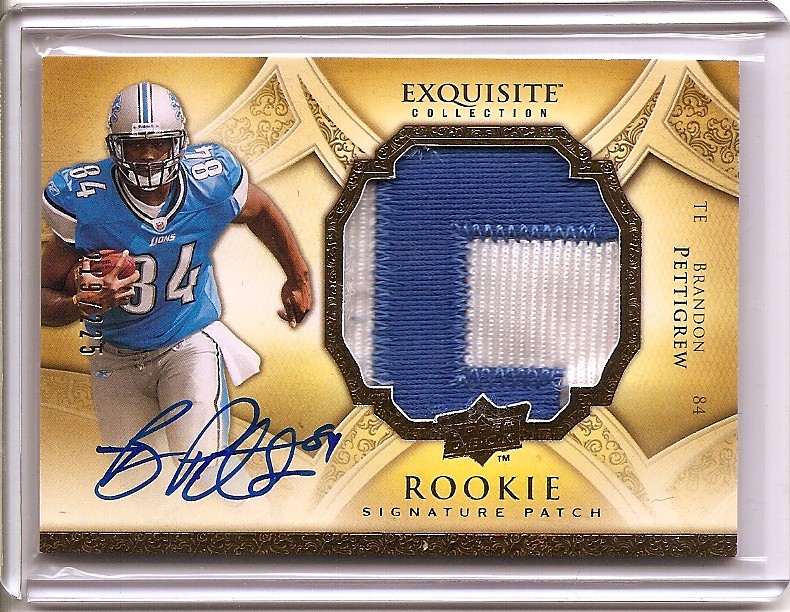The image depicts a highly detailed and meticulously preserved piece of sports memorabilia, specifically an Exquisite Collection Rookie Signature Patch football card of Brandon Pettigrew. The card features a central gold background with the words "Exquisite Collection" prominently displayed. Beneath it, in smaller lettering, the word "collection" is inscribed. On the bottom center, large black letters against a yellow background announce "Rookie Signature Patch," accompanied by Pettigrew's autograph in cursive on the bottom left corner.

The card showcases an image of Brandon Pettigrew, an African American football player, wearing a silver helmet with a face mask, a blue Detroit Lions jersey with the number 84, and holding a football in his right hand across his chest. The player's image occupies the left side of the card, which is situated horizontally, akin to a credit card layout.

The card also features a woven C emblem and a piece of Pettigrew's jersey inlaid into the design, underscoring its status as a valuable collectible. In black letters on the right side, it states "Brandon Pettigrew." Additionally, the card has an embossed number indicating it is 219 out of a limited edition of 225. The card is encased in a protective plastic case, resting on a white surface, enhancing its preservation and display.